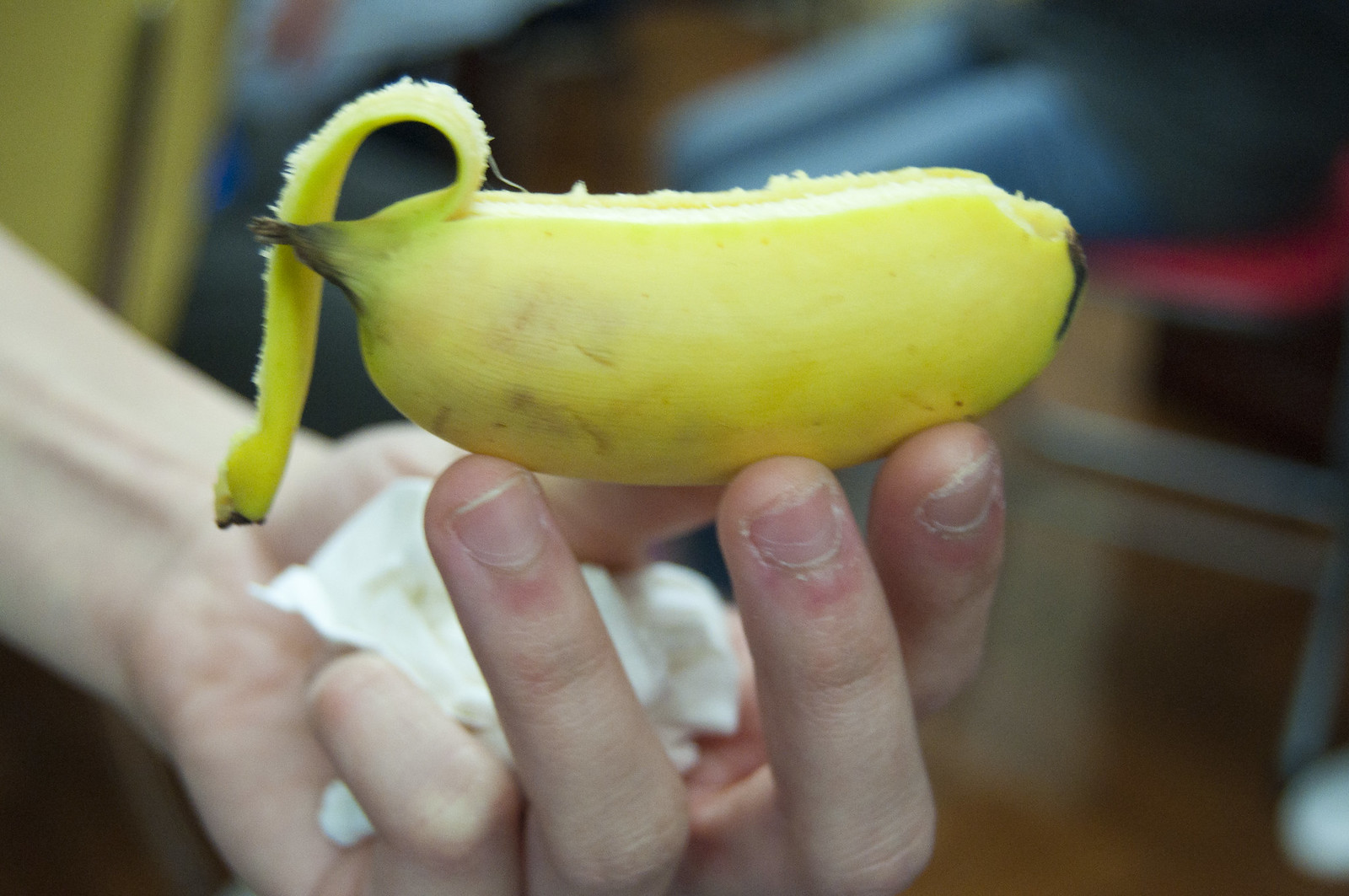A close-up photo captures the delicate details of a person's hand holding a banana against a blurred background, with soft hues of blue, pinkish red, and tan. The hand, with its white skin and slender wrist, appears to belong to a male, possibly a teenager, given the youthful contour and size. The three visible fingers, excluding the hidden pinky and thumb, are curled up, revealing bitten, low-cut nails that are reddish around the edges and somewhat unkempt. Nestled within the cup of the hand is a crumpled white tissue. The banana, ripened to perfection with minimal black spots, is held delicately at the fingertips, slightly tilted to the right, obscuring its length. The tip, bearing a small black mark from where it was severed from the stem, contrasts with the single, slender peel that has been pulled back and gently drapes down towards the wrist, accompanied by a solitary string from the banana’s flesh.